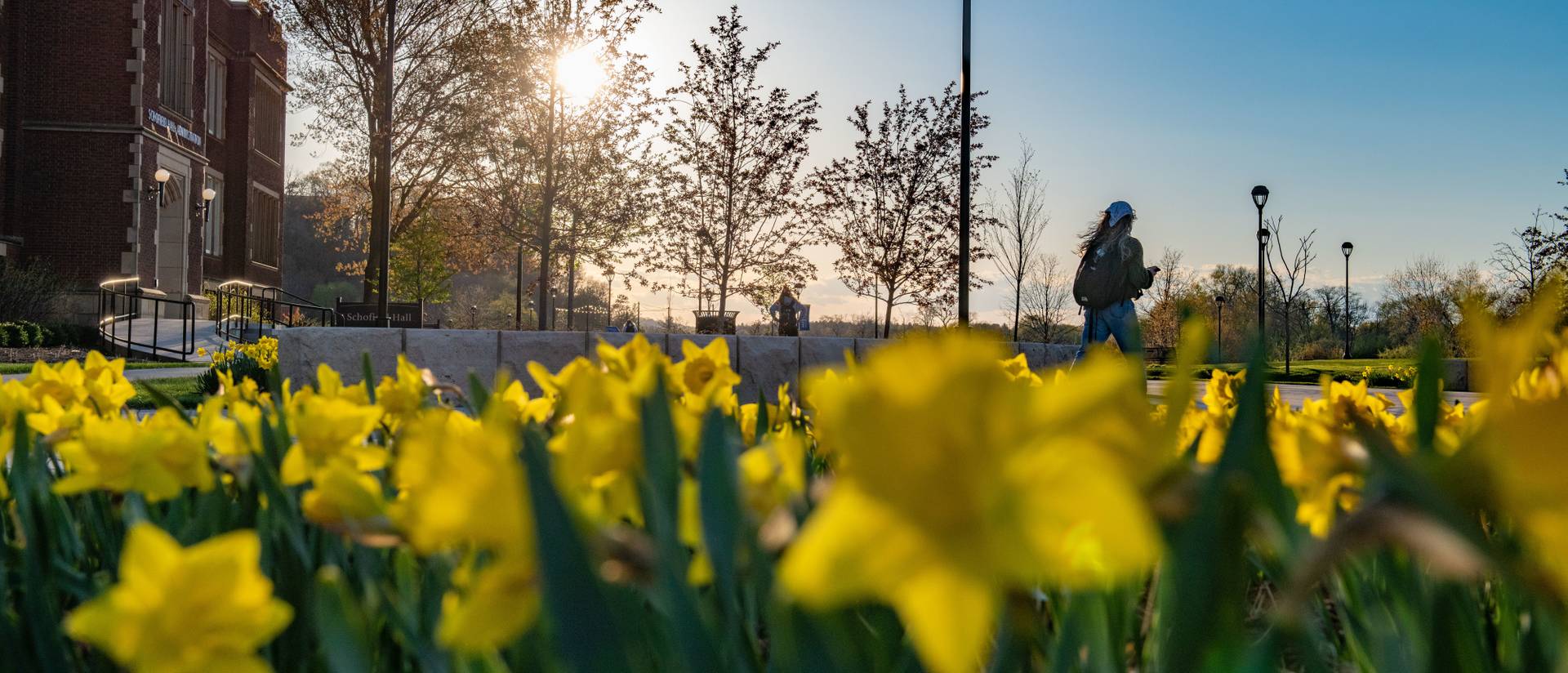The photograph is a horizontally aligned close-up, capturing a vibrant scene at ground level. Dominating the foreground are numerous yellow flowers, slightly blurry up close but becoming more focused toward the middle and upper parts of the image. Each flower, including their centers, is a vivid yellow among tall green grass. In the mid-ground, a woman dressed in jeans and carrying a backpack walks toward the right, seemingly engaged with her phone. Further back, a brown brick building is visible on the upper left, marked by black railings and a ramp. Black street lamps punctuate the scene along with distant trees, some obscuring the sun peeking through on the left side. The clear blue sky stretches across the upper right, framing this beautifully lit morning setting.